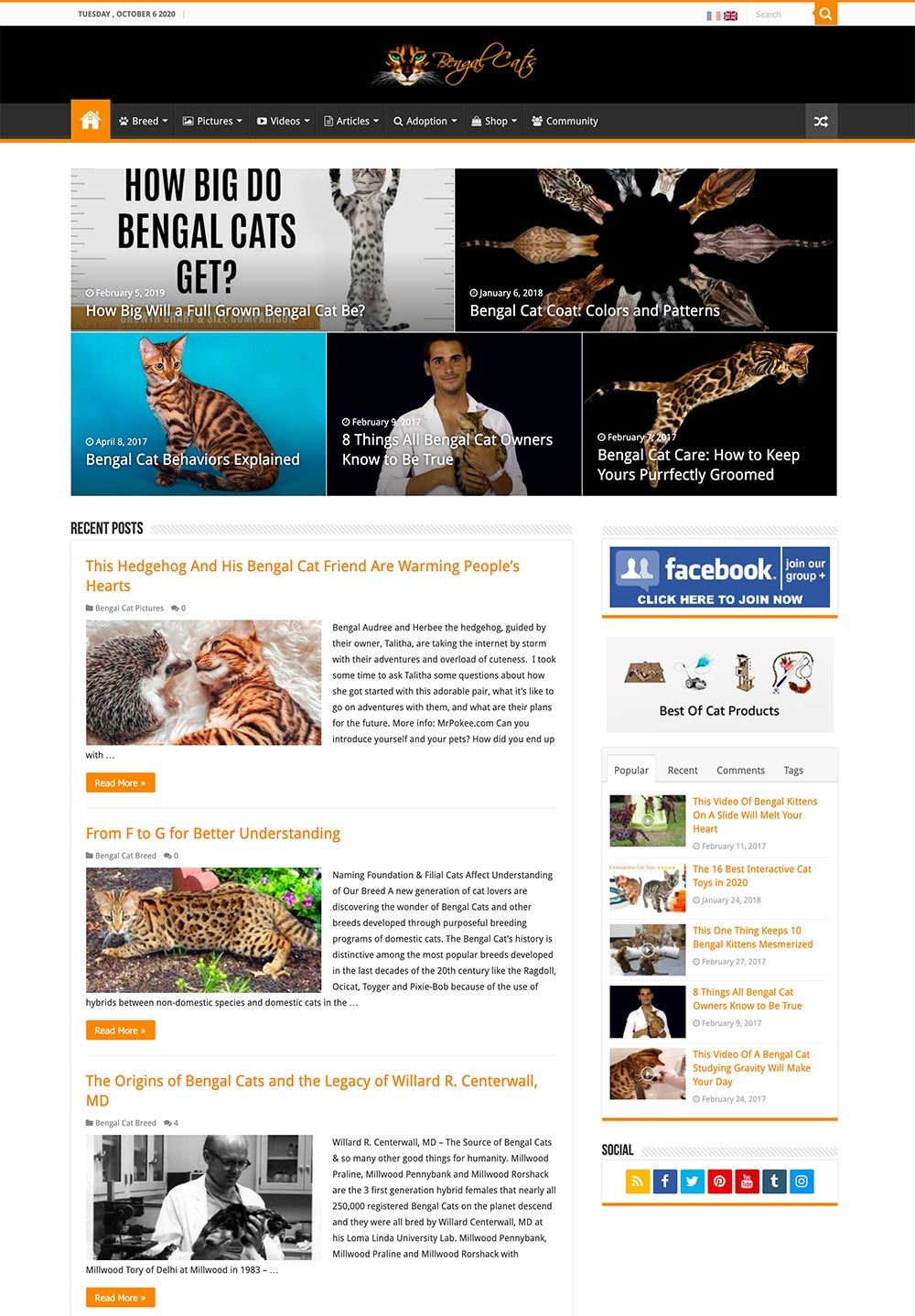The web page titled "Bengal Cats" is an extensive resource filled with various images and information about Bengal cats. At the top of the page, there is a section dated Tuesday, October 6, 2020, featuring clickable links that lead to more detailed content. Topics covered include the size of Bengal cats, their behaviors, and how big they get when fully grown.

The web page also explores the different coat colors and patterns of Bengal cats and offers an article titled "Eight Things All Bengal Cat Owners Know to be True." There are sections dedicated to Bengal cat care, emphasizing methods to keep them perfectly groomed. 

Additionally, the page provides a link to join a Facebook group called "Best of Cat Products," where cat enthusiasts can share and learn about the best products for their feline friends. One of the recent posts highlighted on the site tells the heartwarming story of a Bengal cat named Audrey and her friend Herbie the hedgehog. Guided by their owner, Talitha, this adorable pair is gaining popularity online for their charming adventures and sheer cuteness. An interview with Talitha explores how she came to care for Audrey and Herbie, offering insights into their future plans.

For more information, the page directs readers to MrPokey.com, where they can learn more about Talitha and her pets and even find a section to introduce themselves and their own pets.